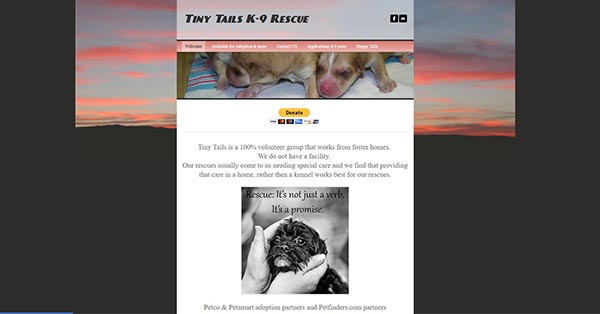In this image, a small screen occupies the center, with the background starting as black on the left and right and transitioning to a light blue sky with orange clouds at the top edges. The central screen displays "Tiny Tails Canine Rescue" in black writing at the top. Below this title are five categories in very small text. The middle section of the screen features a few puppies with light brown and white fur. Further down, there's a prominent yellow button, followed by some very small gray text. At the bottom, there is a black and white picture of a baby black puppy, with the text "It's not just a York, it's a promise" written at the top of the image in black writing. Below the puppy picture is a very small sentence on a white background, completing the composition of the image.